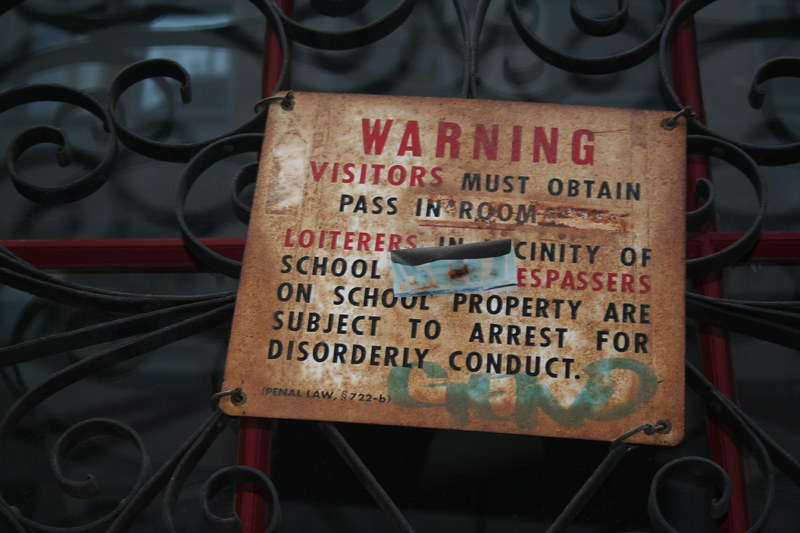This horizontally aligned rectangular photograph captures a weathered and rusted sign attached to an ornate black wrought iron fence, likely part of a gate or protective covering. The sign, once predominantly white, is now largely an orange rust color, with remnants of its original white at the edges. It is secured to the fence with zip ties at each corner. Bold red letters at the top of the sign spell out "WARNING." Below, in smaller black letters, it reads, "VISITORS MUST OBTAIN PASS AND ROOM," with the specific room information scratched out. Beneath that, the message continues, "LOITERS IN VICINITY OF SCHOOL TRESPASSERS ON SCHOOL PROPERTY ARE SUBJECT TO ARREST FOR DISORDERLY CONDUCT." A bent and rusted metal bracket obscures part of the text. The background of the photograph features what appears to be a reflective, dark-colored glass window framed by a black metal grid and red wooden lines. The sign itself shows further aging and wear, with additional graffiti or marks in varying colors, suggesting long-term exposure to the elements and human interference.